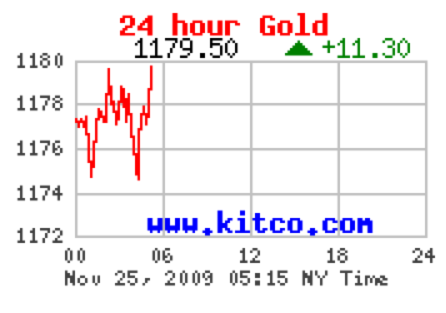The image is a digital line graph titled "24-Hour Gold" in red text at the top. Below the title, it shows a gold price of 1179.50, with a green triangle indicating an increase of 11.30. The y-axis ranges from 1172 to 1180, with intervals at 1172, 1174, 1176, 1178, and 1180. The x-axis represents time in hours, from 0 to 24, marked at intervals of 00, 06, 12, 18, and 24. The red, jagged line on the graph depicts the fluctuating gold price over the 24-hour period, with notable highs and lows. At the bottom of the graph, the date and time stamp "November 25th, 2009, 0515 New York time" is displayed. Additionally, "www.kitco.com" is noted in blue at the bottom left.